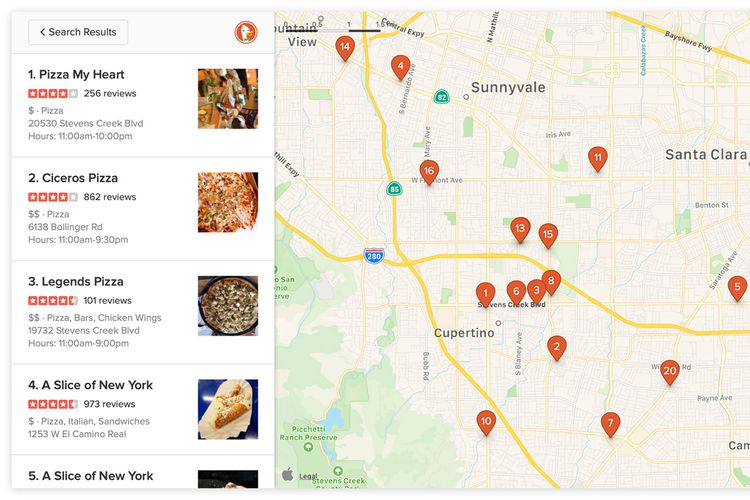The image is a horizontally rectangular screenshot from a Google search results page showing pizza restaurant options. On the left side of the frame, there is a vertical list of pizza restaurants: Pizza My Heart, Cicero's Pizza, Legends Pizza, followed by A Slice of New York listed twice, possibly indicating different locations. The second listing of A Slice of New York is partially cut off, with no additional information visible beneath it. The right two-thirds of the frame displays a map pinpointing the locations of these restaurants, each marked by a numbered icon correlating to the list. Pizza My Heart and Cicero's Pizza, the first two listings, have four-star ratings. Legends Pizza, the third listing, and A Slice of New York, the fourth, both boast four-and-a-half-star ratings.